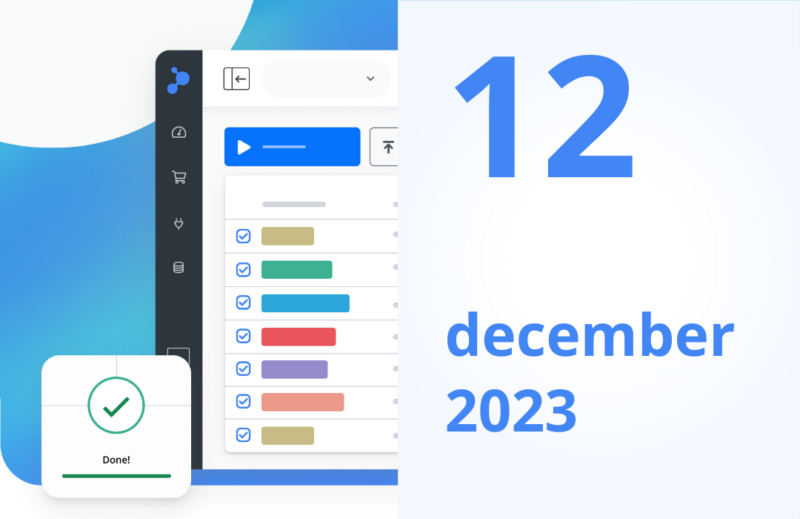The image appears to be a screenshot of a website with a white background. On the left side, the background transitions to blue towards the bottom, while the right side remains predominantly white. Prominently displayed is a large blue number "12" with the text "December 2023" in lowercase blue font beneath it.

The left portion of the screen resembles a calendar interface. At the top left, there's a white circle. Below it is a rectangular area bordered by a black line on the left, featuring various icons including a clock, shopping cart, heart, and calculator.

Adjacent to this area is a section with multiple rows. The top row is blue and includes a play button icon. Below it, there is a row that seems to depict a multicolored graph or chart, with colors including brown, green, blue, red, purple, pink, and another shade of brown. Each color segment is accompanied by a box with a checkmark to its left.

At the very bottom corner of the left segment, there's a white square containing a circle with a green checkmark. Underneath the circle, the word "done!" is displayed with an exclamation mark, and a green line runs beneath it.